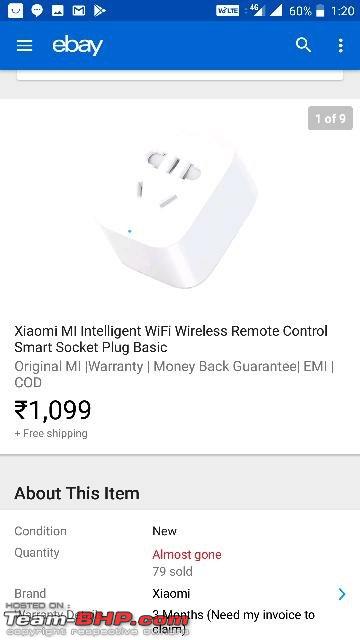This image displays the eBay app on a smartphone screen. At the top, there is a blue header featuring a dark blue line with icons for the Play Store, Gmail, Photos, Tech Chat, and one unidentified app. On the right side of this line, the status indicators include 4G signal bars, LTE connection, a battery level at 60%, and the time displayed as 1:20.

Beneath this, a lighter blue bar contains a hamburger menu on the left followed by the "eBay" logo, a triple vertical dots icon for the additional menu options, and a magnifying glass icon for search. In the main content area, the screen shows "1 of 9" above a product image of what appears to be a smart plug.

The product title reads: "Xiaomi XIAOMI MI Intelligent Wi-Fi Wireless Remote Control Smart Socket Plug Basic." The listing highlights key features including "Original MI Warranty," "Money Back Guarantee," "EMI," and "COD." The price is listed at 1099, presumably in Indian Rupees, accompanied by a note of free shipping.

Below a grey line, additional details about the item are displayed: the condition is marked as "New," the quantity is stated as "Almost Gone" in red, and "79 sold" is noted in brown. The product brand is listed as "Xiaomi," and the warranty mentioned appears to be for 3 months. However, the last couple of lines of text are partly obscured by an overlay of the team-bhp.com logo.